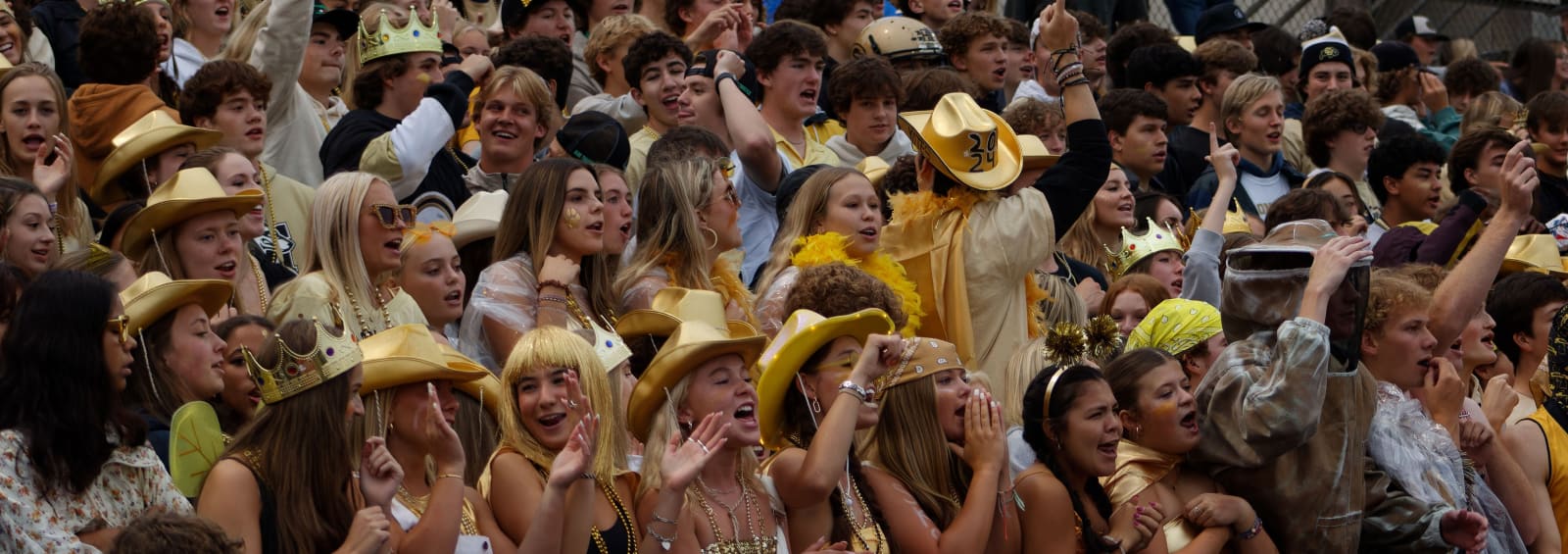An energy-filled panorama captures an enthusiastic crowd, predominantly young women, at what appears to be a college football game. Clad in a vibrant sea of gold-yellow attire, the crowd displays unity through their team colors. Many participants sport distinctive accessories such as yellow cowboy hats, crowns, and bandanas, with several individuals even donning themed outfits like a beekeeping suit, adding to the spectacle. The focus of the front section is on the women, while the men are mostly spotted higher up in the image, creating a layered composition. Arms are raised in fervent support, faces are expressive with cheering, smiling, and shouting, all directed towards the right, capturing the intensity and excitement of the event. Notably, a man in the middle, stands with his back turned, wearing a striking yellow cowboy hat emblazoned with "2024," possibly a nod to an upcoming milestone or graduation year. The scene is a vibrant testament to school spirit and camaraderie among the fans.